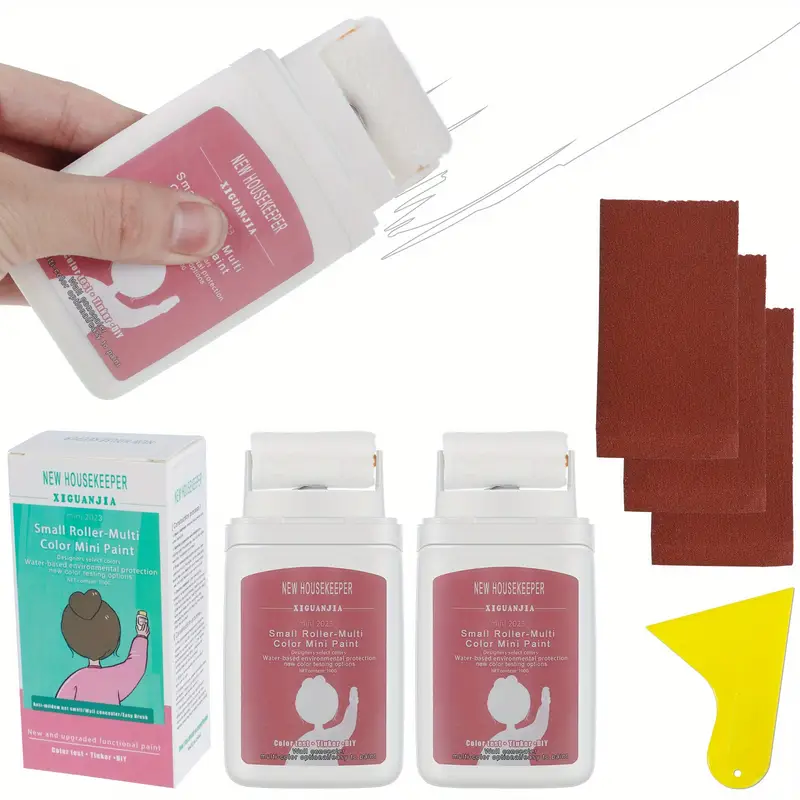This is a detailed photograph of a painting tool set called "Small Roller Multi-Color Mini Paint," made by a brand known as "New Housekeeper," with the product name appearing as "Zinguangya" on the box. The primary box is cyan and pink, labeled with details such as "new and upgraded functional paint" and "color test tinker by Tinker DIY." The main feature is a small white roller that resembles a stick of deodorant but is designed to roll paint onto walls. The product packaging includes an image of a woman in a pink sweatshirt demonstrating the roller, alongside a white silhouette of her on two other paint rollers, also part of the set. In the top left corner, a hand is gripping the roller, showcasing its use. To the right of the main product box, there are also three reddish rectangular strips resembling sandpaper and a yellow scraper for removing paint.